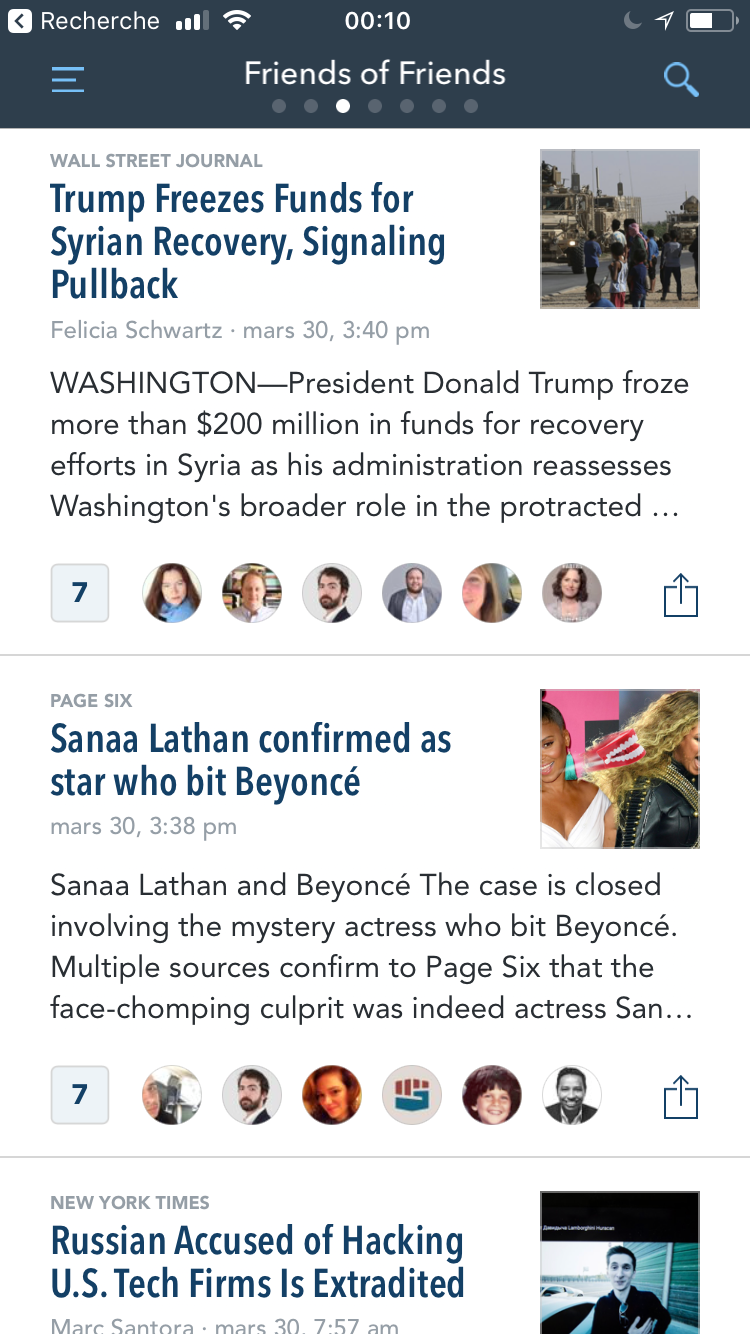### Detailed Caption:

This is a mobile screenshot from a news aggregator site displayed on an iPhone. At the top, the mobile screen features a dark bluish-gray background that includes several status indicators. On the left, a back arrow or triangle bracket inside a white box is followed by the text "Resheri." The status bar shows three out of four cell signal strength bars, full Wi-Fi strength, the current time of 00:10, a crescent moon icon indicating Do Not Disturb mode, a compass navigation arrow, and a battery icon that is about 60% charged.

The screen view confirms it's an iPhone display, indicated by the seven dots at the bottom with the third dot highlighted, representing the selected page, titled "Friend of Friends." To the right of this title is a blue search magnifying glass icon, and to the left are three horizontal lines symbolizing a menu.

Visible articles include two full headlines and part of a third. The first article is from the Wall Street Journal, titled "Trump Freezes Funds for Syrian Recovery, Signaling Pullback," authored by Felicia Schwartz with a timestamp of March 33, 4:40 PM. The thumbnail shows a Syrian street with a military vehicle. The text blurb begins with "Washington, President Trump froze more than $200 million in funds for recovery efforts in Syria as his administration reassesses Washington's broader role in the protracted..." Below this article is a blue box with the number "7" and six circular avatars, along with a share button.

The second article from Page Six is titled "Sanaa Lathan Confirmed as Star Who Bit Beyoncé." It includes a split image: a person on the left and Beyoncé on the right. The text snippet reads, "Sanaa Lathan and Beyoncé, the case is closed involving the mystery actress who bit Beyoncé. Multiple sources confirmed to Page Six that the face-chomping culprit was indeed actress San..." Again, there's the recurring blue box with the number "7" and six avatars, one of which is a sketch of a fist with red fingers and a blue thumb and bottom.

The partially visible third article from the New York Times is titled "Russian Accused of Hacking U.S. Firms is Extradited," authored by Mark Santora, dated March 30th, 7:57 AM.